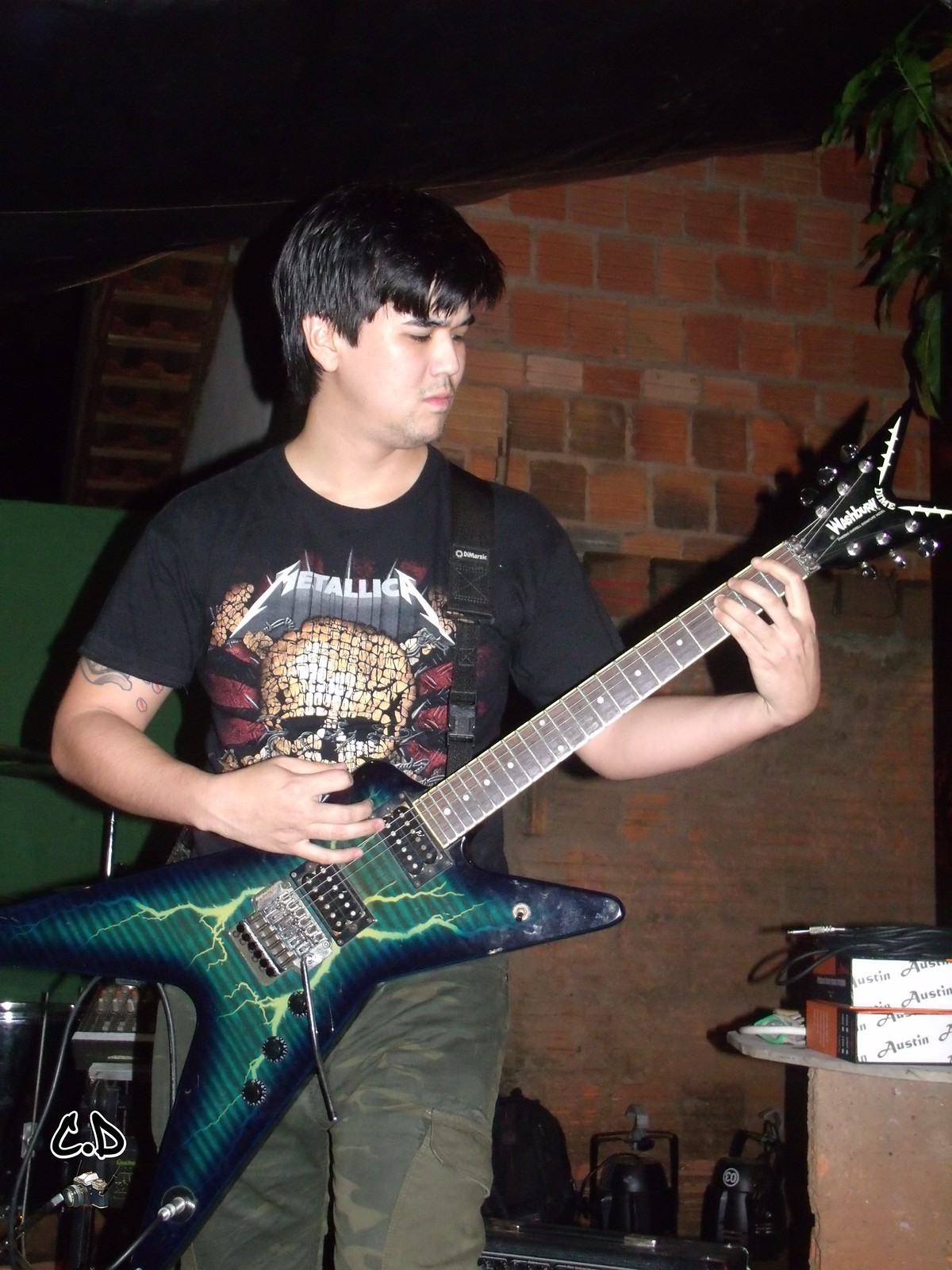The image showcases a black-haired man standing against a rough, red brick wall with varied shades of red, maroon, and brown. He is wearing a black short-sleeve Metallica t-shirt, adorned with the band's logo at the center. Below the logo sits a prominent brown skull surrounded by red stripes. The man sports khaki army pants and visibly has a tattoo. He is holding a distinct green electric guitar with a star-shaped body and sharp spikes at the end. The guitar features an eye-catching paint job resembling green lightning bolts. His guitar appears to be plugged in, with wires extending from it, hinting at its readiness for play. At the bottom right foreground, there's a table cluttered with books and wires, indicative of musician equipment possibly for a stage setup. Notably, the image also has the letters "CD" near the bottom corner, adding a mysterious element to the scene.